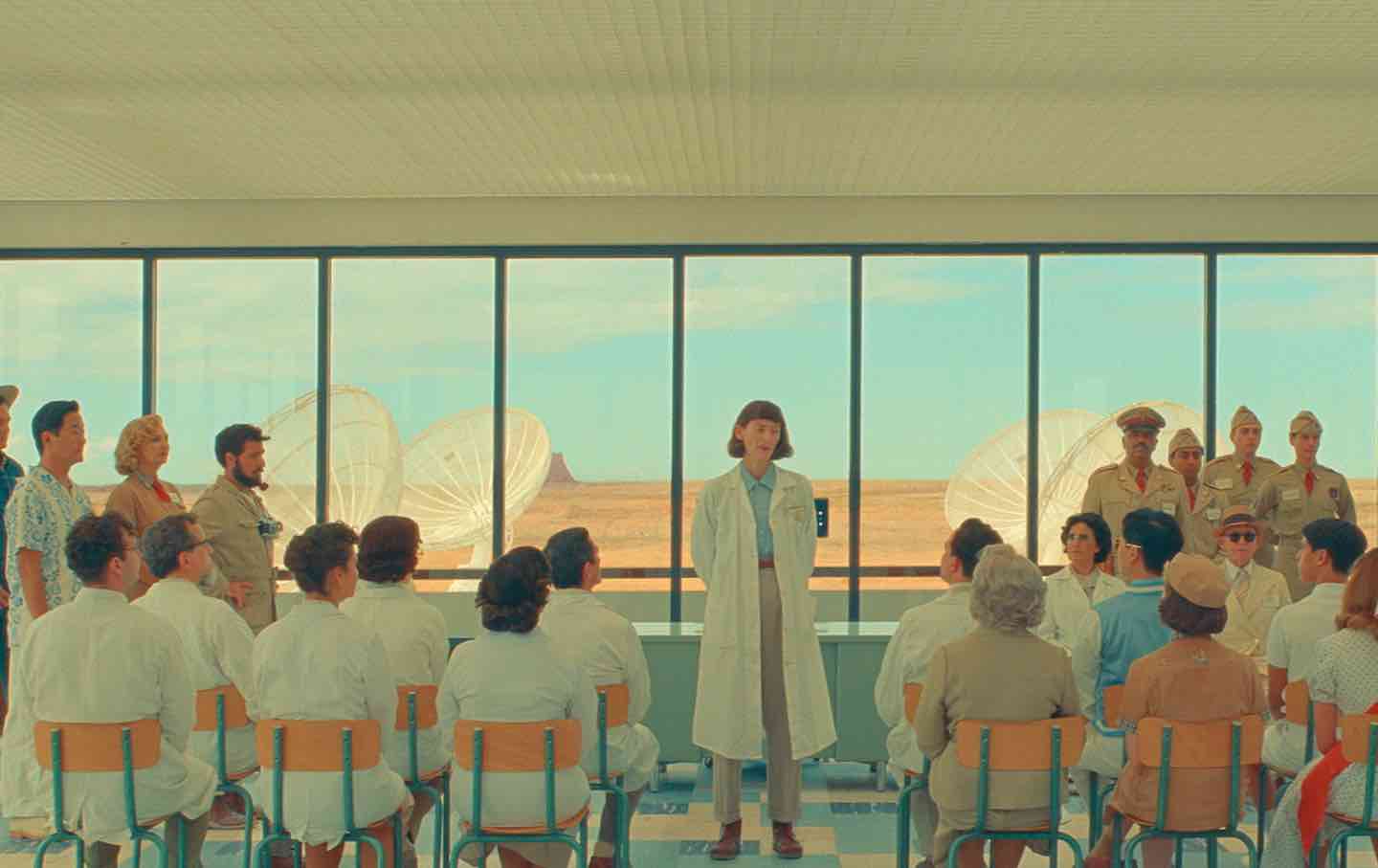In a vintage Norman Rockwell-style illustration, a woman scientist dressed in a long white lab coat, blue shirt, and beige pants stands at the center of a room, giving a presentation to an audience of seated scientists and military personnel. The scientists, also predominantly in white lab coats, sit on metal-framed chairs with wooden seats and backs, their attention fixed on the woman. To the right, four men in khaki military uniforms watch intently. The backdrop is a large glass window revealing a sprawling desert mesa landscape, replete with orange sand and large white satellite dishes pointing skyward, hinting at a likely Arizona location. The woman faces the viewer, adding an engaging dimension to this meticulously detailed, vintage art piece.